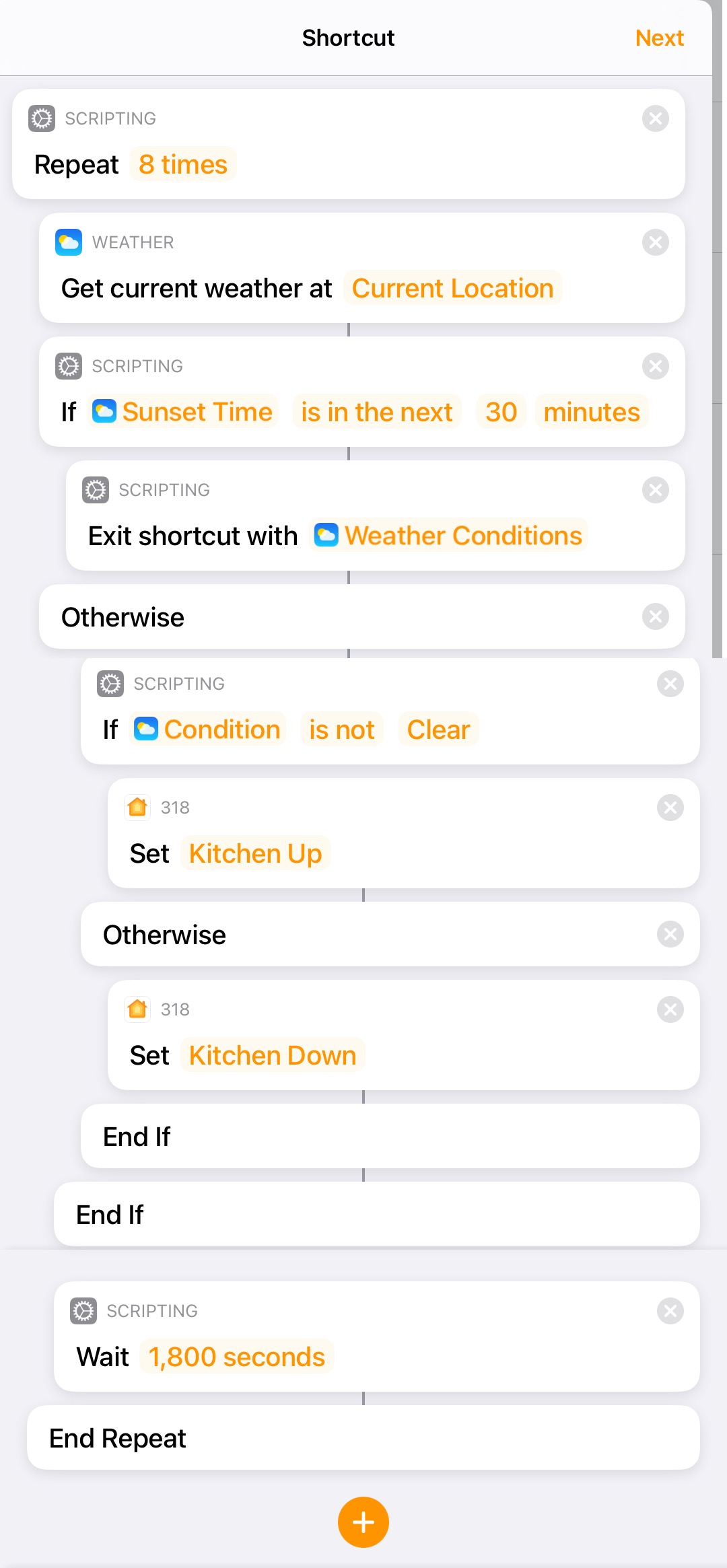This screenshot displays a detailed view of a shortcuts menu for alerts on a mobile phone. The interface features a light gray header at the top, with the word "Shortcuts" centered and "Next" in orange font positioned to the right.

Below the header, the interface is filled with a series of white alert boxes, each accompanied by an "X" on the right for easy removal. The first alert box, labeled "Scripting" in small gray font, details a command to "Repeat 8 times" in orange font.

The next alert box is related to the weather; it displays "Weather" at the top left and, in bold black letters, instructs to "Get current weather at" with "Current Location" highlighted in bold orange font. 

Following this, another scripting command appears, stating: "If weather sunset time is in the next 30 minutes," again in orange font. 

Sequentially, the next scripting box reads "Exit shortcut with weather conditions otherwise," flowing into another scripting box that states: "If condition is not clear."

A subsequent alert, recognizable by an orange house icon on the top left and "318" in small gray letters, includes the instruction: "If can set kitchen up." The next box succinctly states "Otherwise" in bold black font.

Below this, another "318" alert dictates to "Set kitchen down." Two following boxes command to "End if." 

Further down, a scripting command instructs to "Wait 1,800 seconds," culminating in an "End Repeat" command. 

Centrally positioned at the very bottom of the screenshot is an orange circle with a white plus icon, likely for adding new shortcuts or alerts.